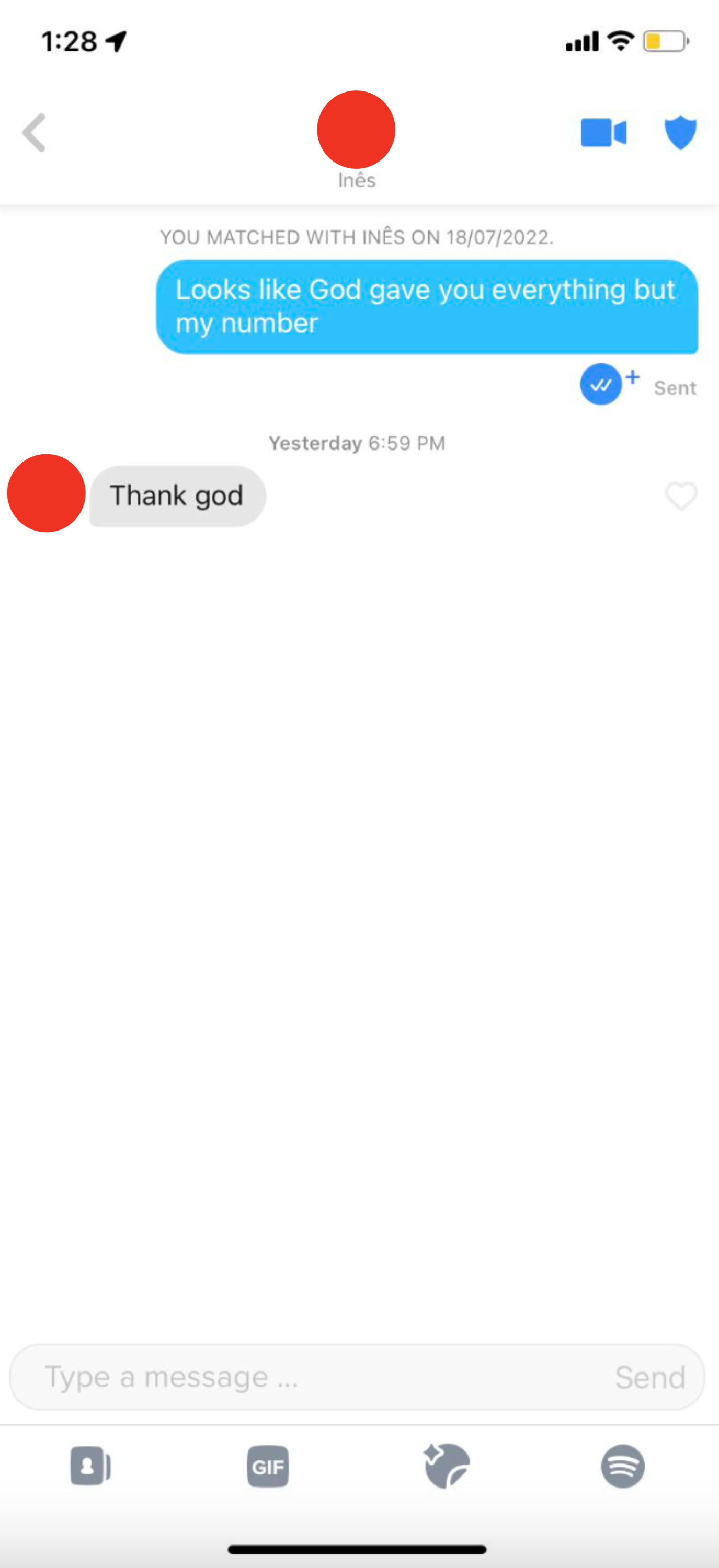This screen capture from an iPhone displays a brief conversation within a dating app. At the top of the screen are the standard iPhone status icons showing the time (1:28), battery level, and signal strength. The usual icons are also present at the bottom of the screen.

The conversation is between the user and a match named INES, with the match notification stating, "You're matched with INES on 18/07/2022." The dialogue begins in a blue text box from the user, saying, "Looks like God gave you everything but my number." Below this message, a timestamp indicates it was sent "yesterday at 6:59 p.m." INES replies in a gray text box, "Thank God," with a small red dot to the left of the text.

Additionally, at the very top of the screen, there's a red dot indicating a new notification. In the upper right corner, two icons are visible: a blue logo shaped like a shield and another shaped like a camera.

The screenshot captures a light-hearted exchange where the user humorously notes the absence of a phone number in their match's profile, and the match cheekily replies with gratitude.